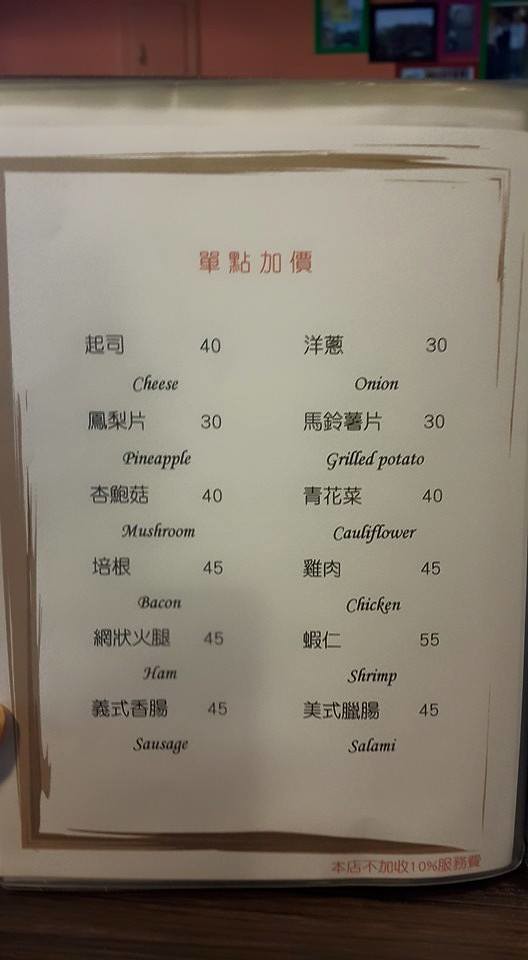The image depicts a page from an Asian restaurant menu. At the top center of the page, there are four Asian characters rendered in a reddish-orange hue. Below these characters, the menu is organized into two columns, listing food items in both English and Asian characters with their respective prices. The first column includes: 

- Cheese: 40
- Pineapple: 30
- Mushroom: 40
- Bacon: 45
- Ham: 45
- Sausage: 45

The second column lists:

- Onion: 30
- Grilled Potato: 30
- Cauliflower: 40
- Chicken: 45
- Shrimp: 55
- Salami: 45

The background of the menu page is white with a subtle border created using brown brush strokes of varying thicknesses, with the right edge showing noticeably less brown.